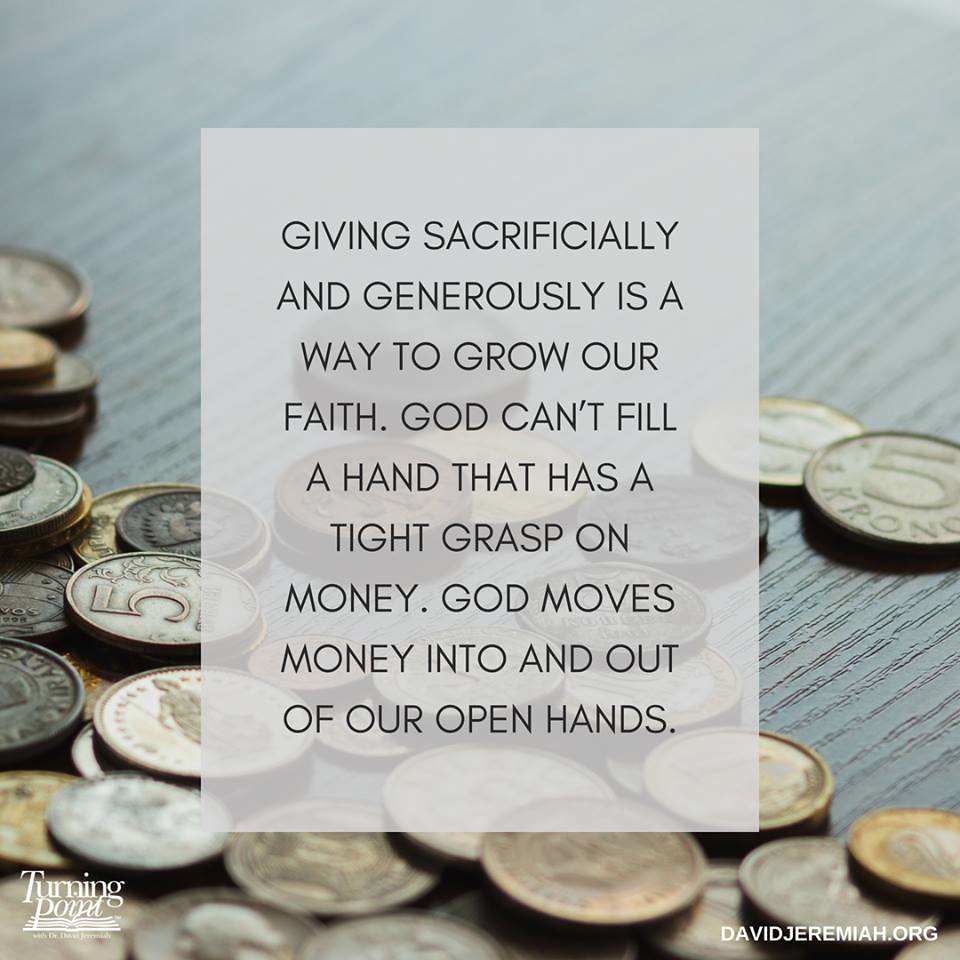The image is an inspirational graphic featuring an array of vintage, foreign coins scattered on a dark, grain-marked wooden table. The coins, primarily five-cent pieces and crone eggs, are mostly concentrated in the lower half of the image, with some in sharp focus in the foreground. Overlapping this backdrop, in the center, is a semi-transparent gray rectangle containing a motivational message in uppercase, thin black font: "Giving sacrificially and generously is a way to grow our faith. God can't fill a hand that has a tight grasp on money. God moves money into and out of our open hands." In the bottom left corner, there’s a logo of an open book next to the words "Turning Point," and in the bottom right corner, the URL "davidjeremiah.org" is displayed in white text.